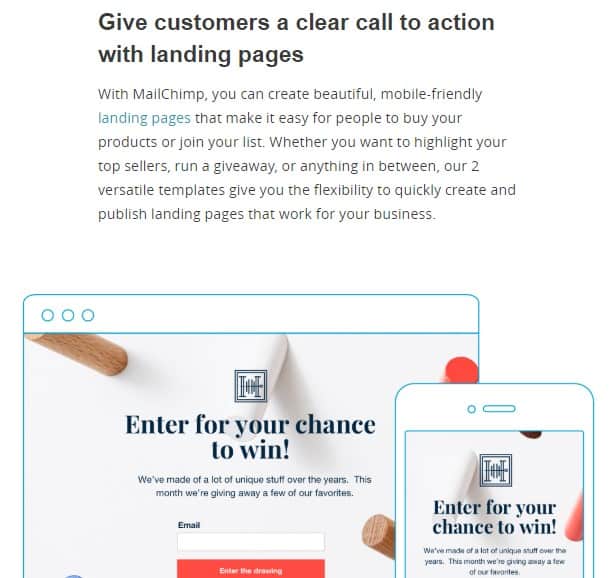The image features a white background with bold black text that reads: "Give customers a clear call to action with landing pages." Below this, in a lighter black font, it says: "With MailChimp, you can create beautiful, mobile-friendly landing pages," with the phrase "mobile-friendly landing pages" highlighted in blue. The text continues to explain that MailChimp's landing pages make it easy for people to buy products or join a mailing list and mentions the flexibility offered by two versatile templates, ideal for various purposes like highlighting top sellers or running giveaways.

In the image, there are two devices displayed: a computer and a smartphone. 

- On the computer screen, there is text that reads: "Enter for your chance to win. We've made a lot of unique stuff over the years. This month we're giving away a few of our favorites," followed by a label "Email" in black next to a white input box for entering an email address. Below the input box, there is a red button labeled "Enter the drawing."

- The smartphone screen shows a similar interface but it is cropped to display only up to where the email address input field is visible, demonstrating the contest entry form on a mobile device.

The image effectively showcases how MailChimp’s landing pages function across both desktop and mobile platforms while providing a specific example of how to create an engaging and actionable giveaway entry form.